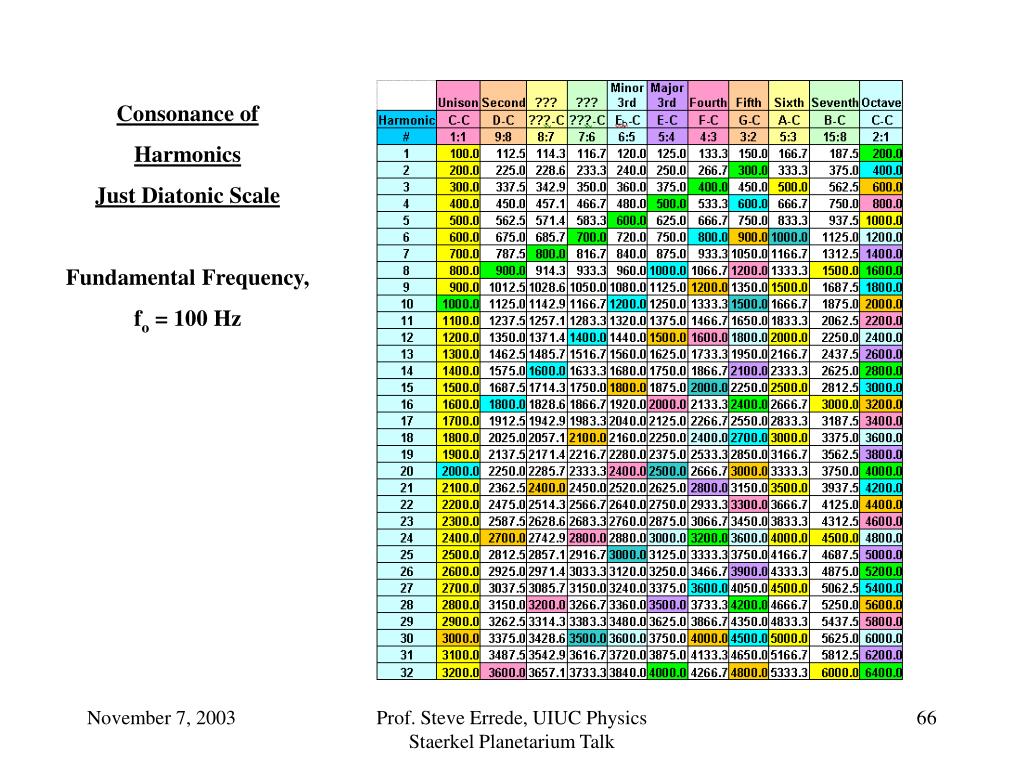This detailed diagram appears to be from a planetarium talk given by a physics professor, specifically Professor Steve Araday of UIUC Physics, on November 7, 2003, at the Starkle Planetarium. The title of the diagram reads "Consonants of Harmonics, Just Diatonic Scale." This intricate chart likely comes from a physics textbook, depicting various harmonics for minor and major scales across 32 numbered rows under a column labeled "Harmonic." Each cell within these rows contains numbers in black font, with some cells shaded in a variety of colors such as green, blue, orange, pink, teal, and yellow, but not all the cells are color-coded, and it’s unclear what the shading signifies. Additional text positioned to the left of the table indicates “Fundamental Frequency, F0 = 100 Hertz.” Text at the bottom notes "Professor Steve Araday, UIUC Physics, Starkle Planetarium Talk," and in the lower left corner, the image is dated "November 7, 2003." The diagram is detailed and multicolored, adding a visual complexity that suggests it’s an educational resource.